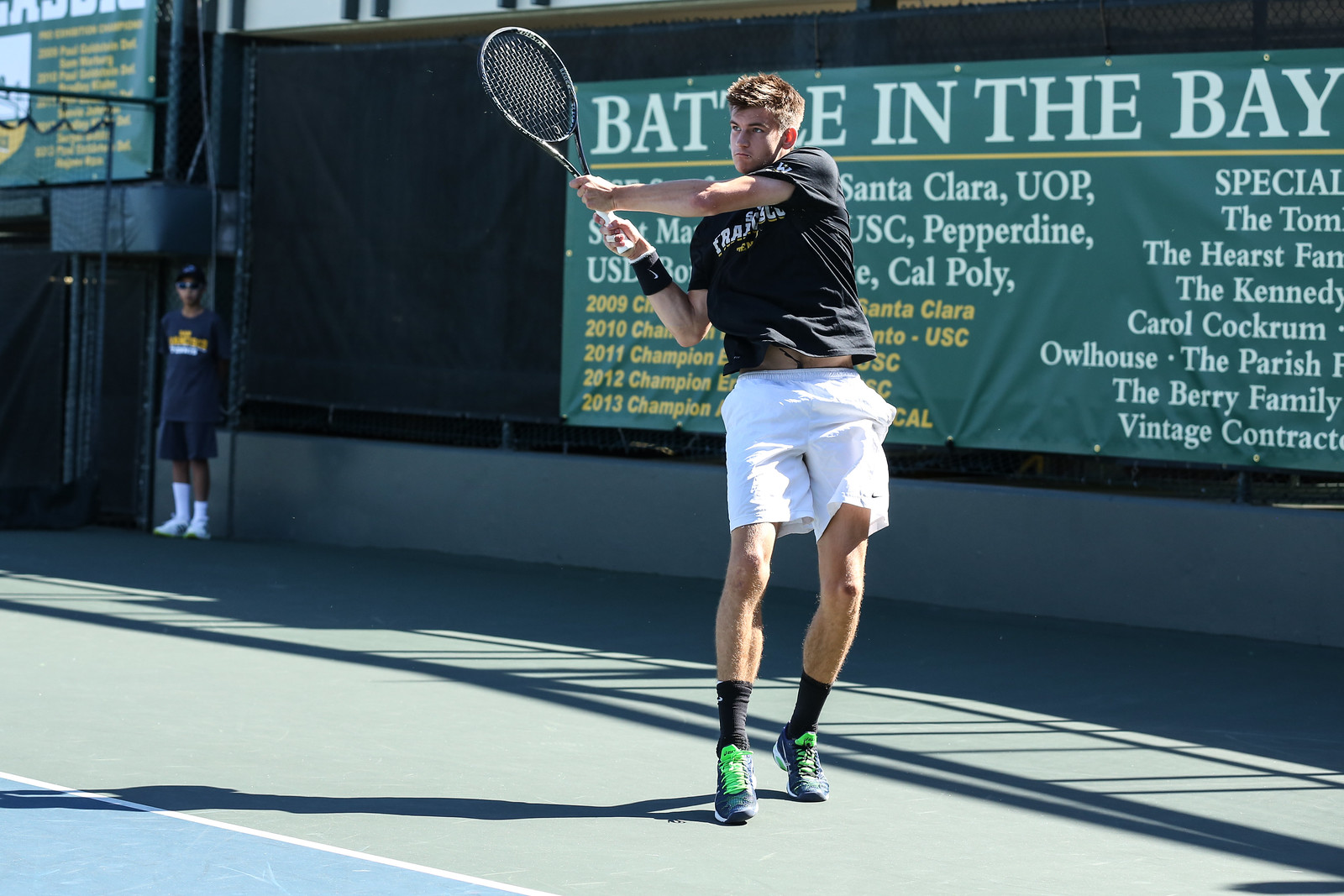The image captures a dynamic moment of a young man playing tennis on a sunny day. He is mid-action, having just hit the tennis ball, with his black racket raised and pulled back on his left side. He is dressed in a black shirt with a partially obscured white logo, white shorts, black socks, and dark tennis shoes featuring light green laces. The backdrop reveals a deep green sign with bold white text proclaiming "Battle in the Bay," along with a mixture of yellow and white text listing different schools, sponsors, and championship years from 2009 to 2013. To the right, partially obscured, additional text includes names such as "the Tom the Hearst family," "the Kennedy," "Carol Cockrum," "Owlhouse," "the Parish," "the Berry family," and "Vintage Contract." In the far left background, a spectator or possibly an official dressed in a dark blue t-shirt, jean shorts, white socks, white tennis shoes, and sunglasses stands near a chain-link fence. A referee, clad in a black hat, black shirt, black pants, and white shoes, is positioned in the corner, observing the match. The court's surface is green, with shadows cast on the floor, and a cropped glimpse of a blue tennis field is visible at the bottom left of the image.